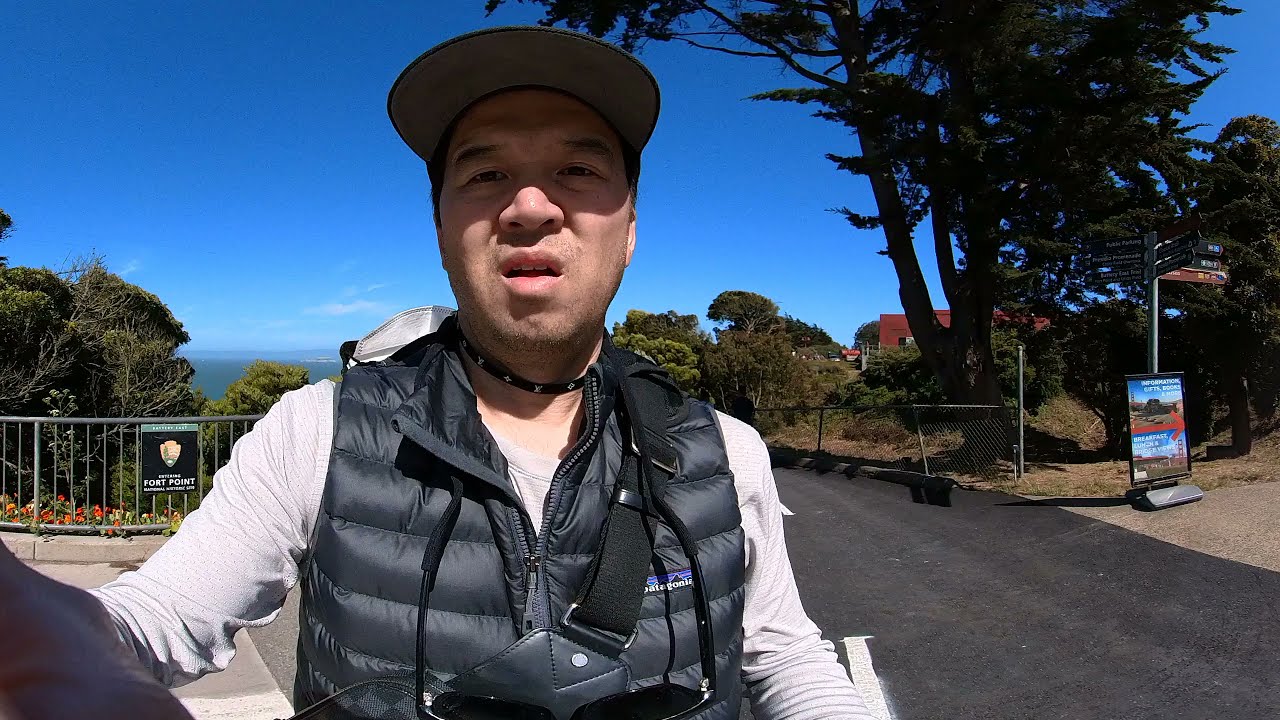In this picture, a man is taking a selfie, seemingly about to go on a hike in Hawaii. He is wearing a black puffy vest over a white long-sleeve shirt, a black baseball cap with a gray rim, and a tight black dog collar necklace. Sunglasses dangle from around his neck. He has olive skin, dark eyes, and a wide nose, with his mouth slightly open revealing his top row of teeth. 

The backdrop includes lush greenery and a picturesque, clear blue sky with no clouds. Behind him to the left, there is a guardrail with a sign that reads "Fort Point," a body of water, shrubs, and trees. To his right, a paved road and a driveway with a fence are visible, along with a pole displaying several directional signs. In the distance, a house with a red roof and other buildings can be seen, contributing to the laid-back, vacation atmosphere of the scene.